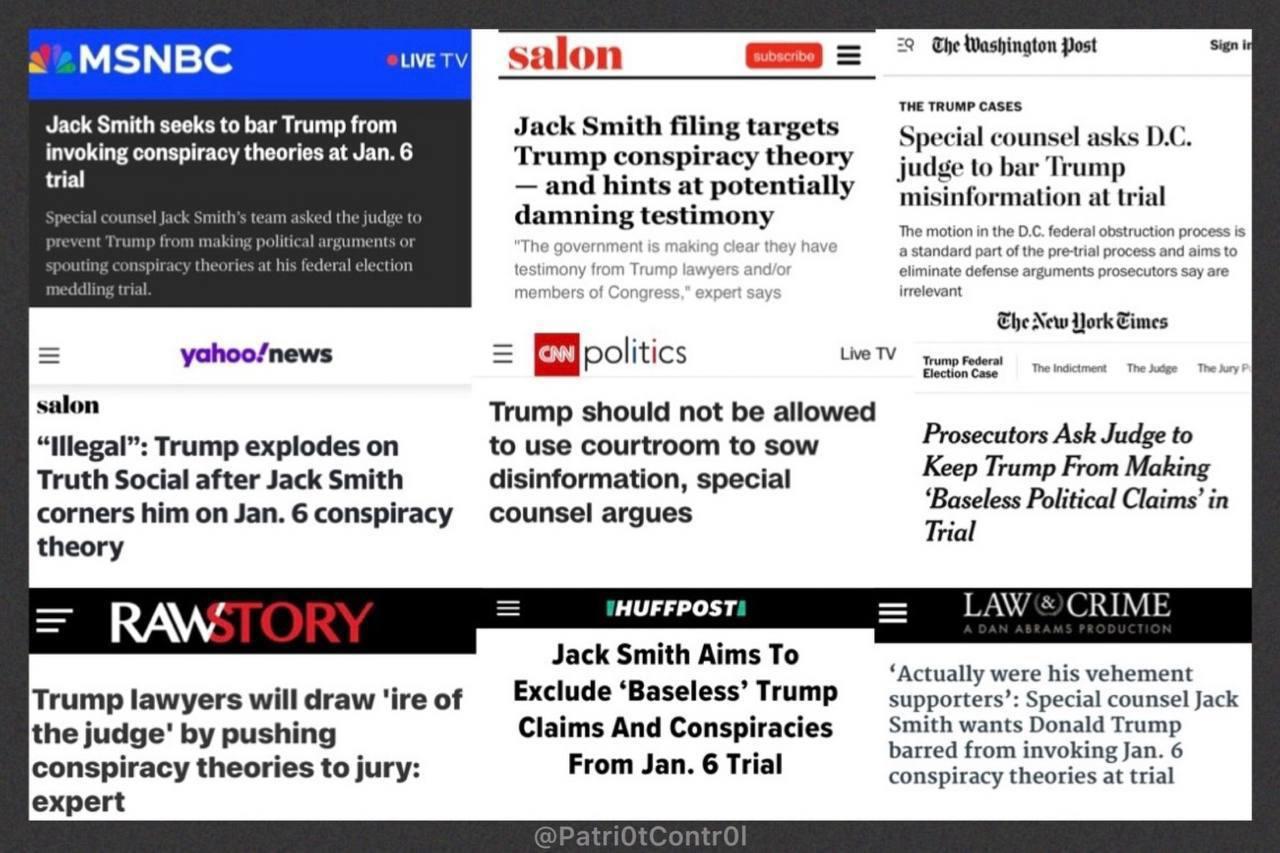This image displays an aggregate view of multiple social media pages and news articles, each focusing on the legal proceedings involving former President Donald Trump and his potential involvement in the January 6th insurrection. In the top left corner, the MSNBC logo is prominently featured with a "Live TV" tag adjacent to it. Beneath MSNBC, there's a headline stating, "Jack Smith seeks to bar Trump from invoking conspiracy theories at January 6 trial," followed by a paragraph providing further details.

On the right side of the MSNBC section, "Salon" is marked, accompanied by a subscribe button and a hamburger menu icon. Below this row, a headline reads, "Jack Smith filing target Trump conspiracy theory hints at potential damning testimony."

Adjacent to this is a fragment of a Washington Post article with the headline, "Special counsel asks DC judge to bar Trump misinformation at trial." Farther to the right, a Yahoo News article is highlighted with the attention-grabbing title, "Trump explodes on social after Jack Smith corners him on January 6 conspiracy theory."

Also visible is an article from CNN Politics and a segment that indicates it's from the New York Times, with a highlighted section titled, "Trump federal election case." On the left-hand side, there's a Raw Story section with "Raw" displayed in white and "Story" in red font. Additionally, content from the Huffington Post and an article from Law & Crime can be seen, both sharing information on the same overarching story. The complex collage of articles underscores the widespread media coverage and the gravity of the legal implications surrounding the events of January 6th.